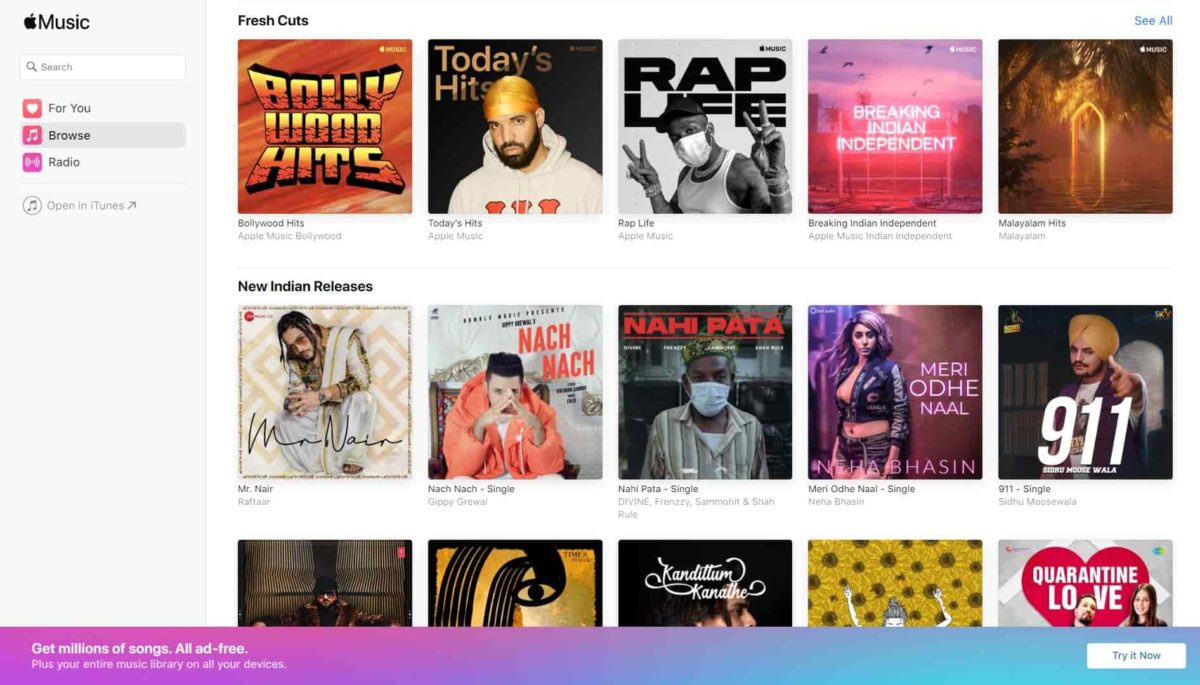This screenshot captures an interface view of the Apple Music application displaying a curated selection of music. The horizontal image frame features the Apple Music logo positioned in the upper left corner, enclosed within a light gray, vertically rectangular window. Directly below the logo, there is a searchable field, followed by a vertical menu listing options labeled "For You," "Browse," and "Radio."

The remainder of the frame is filled with various square album covers and playlist icons, indicating different music listings. Centrally positioned at the top of the interface, a bold heading reads "Fresh Cuts," immediately followed by a row of horizontally aligned, square images depicting the latest music selections. These include categories such as "Bollywood Hits," "Today's Hits," "Rap Life," "Breaking Indian Independent," and "Malaysian Hits," although some text may be challenging to read due to its small print.

Beneath the "Fresh Cuts" section lies another highlighted heading, "New Indian Releases," featuring a collection of recently released tracks. Featured in this listing are the albums and singles: "Mr. Nair," "Knock Knock Single," "Nahi Pata Single," "Mary Odehnal Single," and "9-1-1 Single." Each cover image is vivid and distinct, ensuring easy recognition of popular and emerging music titles curated by Apple Music.